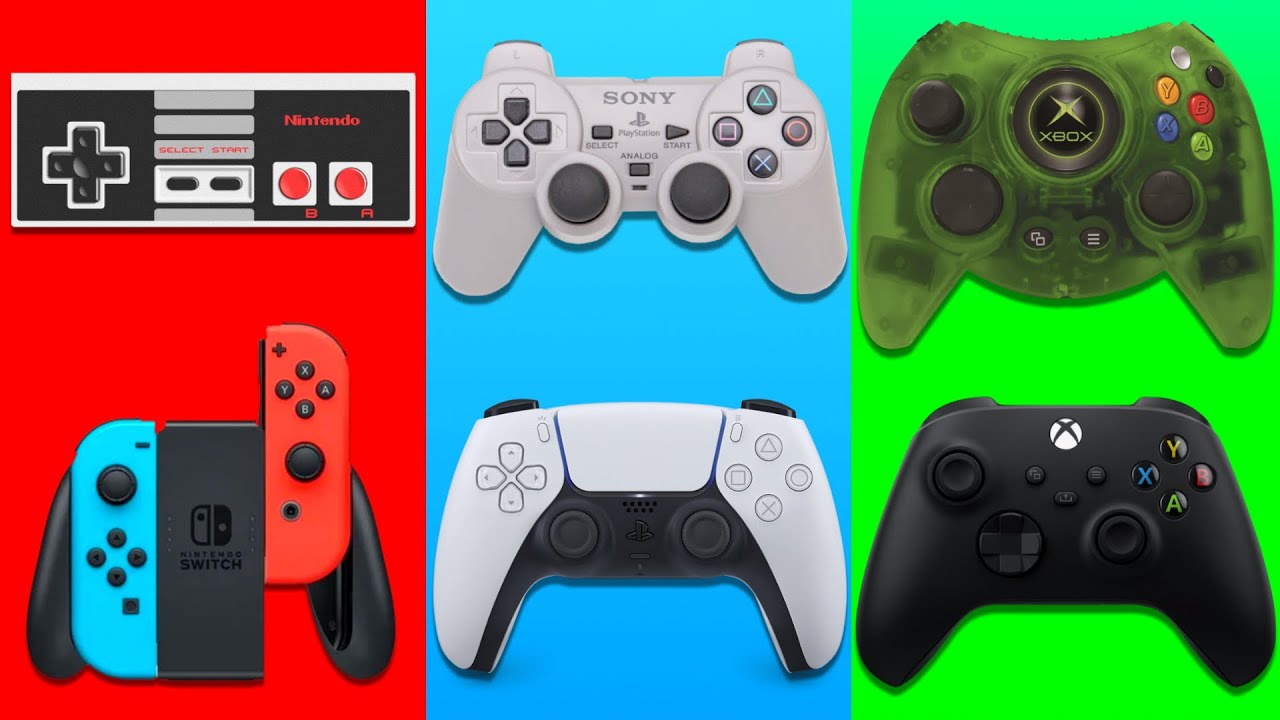This photograph showcases the evolution of various gaming controllers across three colorful columns. On the left, set against a red background, are the Nintendo controllers. At the top is the iconic original Nintendo controller, a boxy device featuring two red buttons labeled "A" and "B," a black square D-pad with four directional arrows, and two small oblong start and select buttons. Below it is the Nintendo Switch controller, split into two parts with a blue section on the left and a red section on the right, each part equipped with four buttons and a joystick.

In the middle column, against a bright blue background, are the Sony PlayStation controllers. Starting with the original Sony PlayStation controller, it’s a light gray device featuring all the familiar buttons: four directional buttons on the left, four shape buttons on the right, and two joysticks at the bottom. Below this is the PlayStation 5 controller, an updated version that retains a similar layout but with a sleeker design.

On the right, set against a neon green background, are the Xbox controllers. The original model showcases a translucent green casing with four colorful buttons—blue, red, green, and yellow—alongside two joysticks. The newer Xbox controller is more compact and made of solid black material but maintains the familiar button configuration with colored action buttons.

This detailed image not only highlights various gaming consoles but also contrasts older models with their modern successors, giving a visual representation of the advancements in gaming technology.